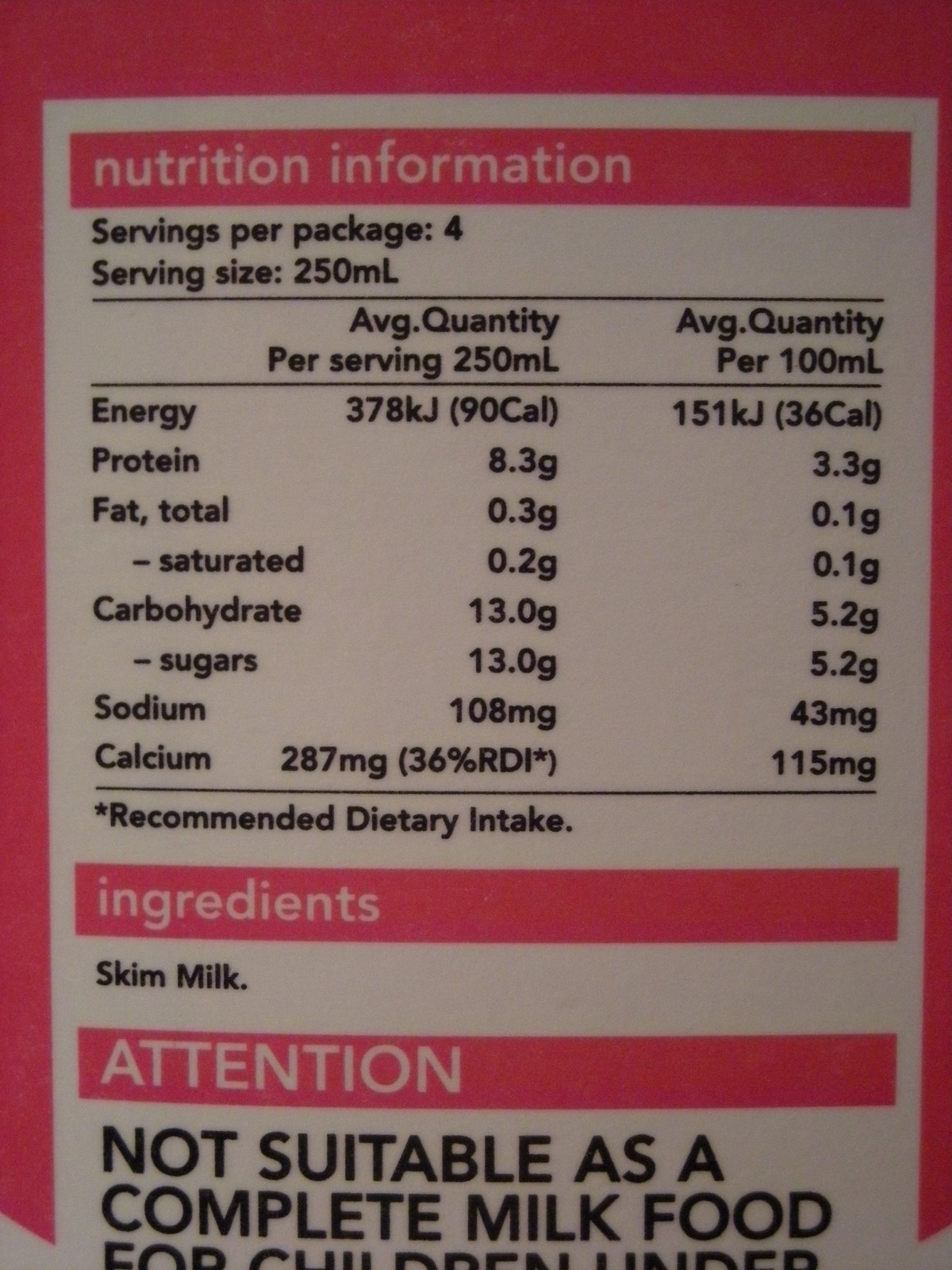The image displays a nutrition label for a product whose primary ingredient is skim milk. The label indicates that there are four servings per package, with each serving size being 150 milliliters. It provides standard nutritional information, listing the amounts of macronutrients typically found in such products. Additionally, there is a section detailing the recommended dietary intake. Towards the bottom of the label, it includes a cautionary note stating, "Attention: Not suitable as a complete milk food for children under," but the statement cuts off, implying that it advises against using this product as a substitute for breast milk for young children. The entire label is set against a pinkish-red background.